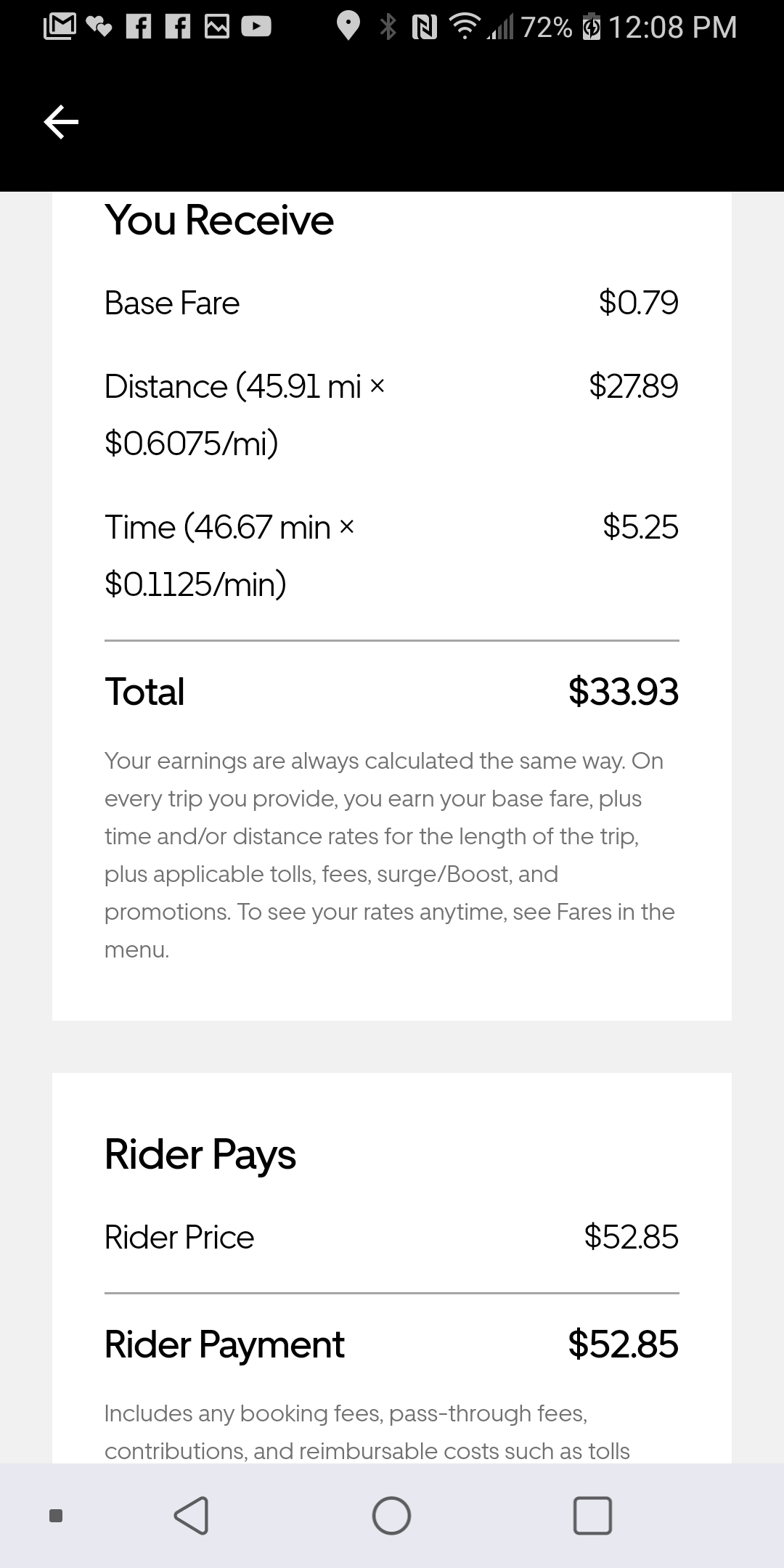A smartphone screen displays a Gmail notification at the top. Below it, a series of icons and text clutter the display, including references to CTNPN, NFC status, WiFi signal at 72%, battery percentage, and a notification from the Telfa APM app. A black bar hosts various icons: a left arrow, USB icon, and more, with an app called Basefer showing a cost of $0.79. The screen also displays distance data of 45.91 miles, calculations involving time and monthly charges, equating to figures like $7.89, $33.93, and earnings per month. Various fare calculations are highlighted, indicating base fares, time and distance adjustments, applicable tolls and fees, promotions, and payment processing fees. The fragmented visual description is concluded with shapes like a square, sideways triangle, circle, and another square positioned at the right-hand side of the screen.